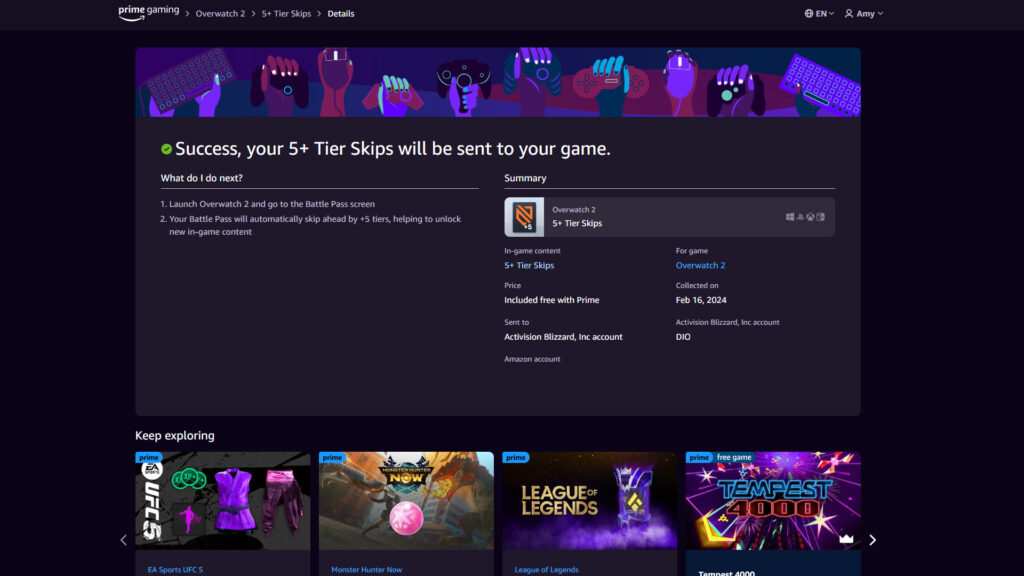Caption: 

This screenshot showcases the Prime Gaming website. At the top left corner, the "Prime Gaming" name and logo are prominently displayed in white. Adjacent to this, the text reads "Overwatch 2, 5+ tierskips", followed by the word "Details" highlighted in bright white. On the top right, there is a profile icon labeled "Amy", and to its left, the letters "EN" accompanied by a globe icon indicate language settings.

The central portion of the image features a confirmation message stating: "Success, your 5+ tierskips will be sent to your game," accompanied by a green checkmark in a circle. Above this, a rectangular inset contains artwork depicting hands holding controllers, suggesting a gaming context.

To the right, the word "Summary" is visible, beneath which is a box labeled "Overwatch 2, 5+ tierskips". On the left, under the header "What do I do next?" with an underlined horizontal line, the instructions are listed:
1. Launch Overwatch 2 and navigate to the battle pass screen.
2. Your battle pass will automatically skip ahead by 5 tiers, aiding in unlocking new in-game content.